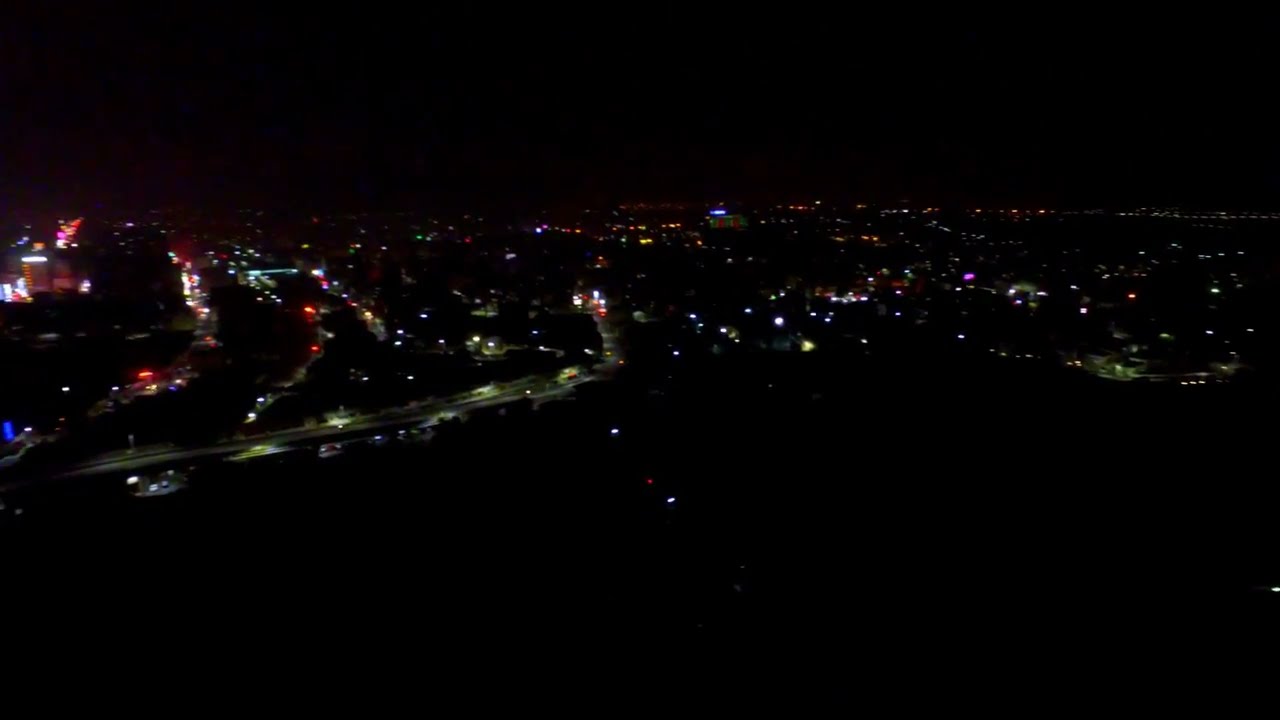The image captures a distant nighttime view of an urban cityscape, likely taken from a high vantage point such as a drone or the rooftop of a tall building. There's a dominant presence of blackness, highlighting the depth of night. The bottom and top sections are enveloped in darkness, only sparingly punctuated by lights, creating a stark contrast against the city lights that cluster in the middle. The left middle part of the image features a roadway with minimal traffic. The lights, scattered and varied in color—ranging from warm yellows and reds to cooler blues and purples—illuminate patches of buildings and streets, albeit in a somewhat subdued manner. The overall scene is not overly dramatic but presents a quiet, mild ambiance, with no readable signs or text and an array of colored lights providing a muted luminescence against the dark urban sprawl.